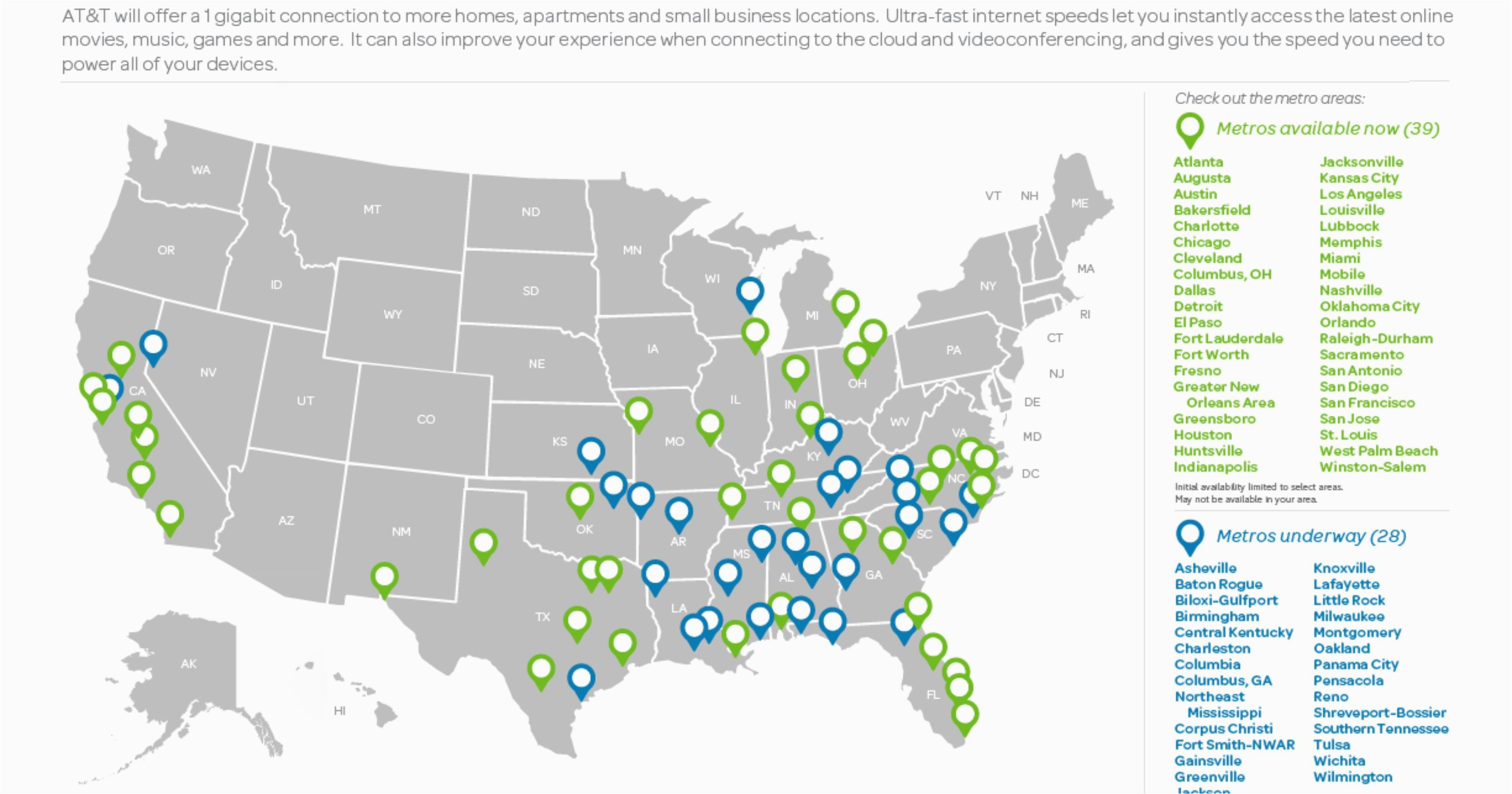This image features a section of a website with a light grey background. At the top of the page, a prominent message from AT&T announces their plan to offer one gigabyte internet connections to more residences, apartments, and small business locations. This ultra-fast internet service promises instant access to online movies, music, games, and more. It also aims to enhance user experiences with cloud services and video conferencing, providing the necessary speed to support multiple devices.

Below the message, there is a map of the United States adorned with blue and green accent points. These points are represented as white circles with either blue or green outlines. According to the map, the green points indicate 39 metro areas where the one gigabyte connection is already available, including:

- Atlanta
- Augusta
- Austin
- Bakersfield
- Charlotte
- Chicago
- Cleveland
- Columbus, Ohio
- Dallas
- Detroit
- El Paso
- Fort Lauderdale
- Fort Worth
- Fresno
- Greater New Orleans Area
- Greensboro
- Houston
- Huntsville
- Indianapolis
- Jacksonville
- Kansas City
- Los Angeles
- Louisville
- Lubbock
- Memphis
- Miami
- Mobile
- Nashville
- Oklahoma City
- Orlando
- Raleigh-Durham
- Sacramento
- San Antonio
- San Diego
- San Francisco
- San Jose
- St. Louis
- West Palm Beach
- Winston-Salem.

The blue points signify metro areas where the service is underway, totaling 28 locations, such as:

- Asheville
- Baton Rouge
- Biloxi Gulfport
- Birmingham
- Central Kentucky
- Charleston
- Columbia
- Columbus, Georgia
- Northeast Mississippi
- Corpus Christi
- Fort Worth-NWAR
- Gainesville
- Greensville
- Jackson
- Knoxville
- Lafayette
- Little Rock
- Milwaukee
- Montgomery
- Oakland
- Pensacola-Reno
- Shreveport-Bossier
- Southern Tennessee
- Tulsa
- Wichita
- Wilmington.